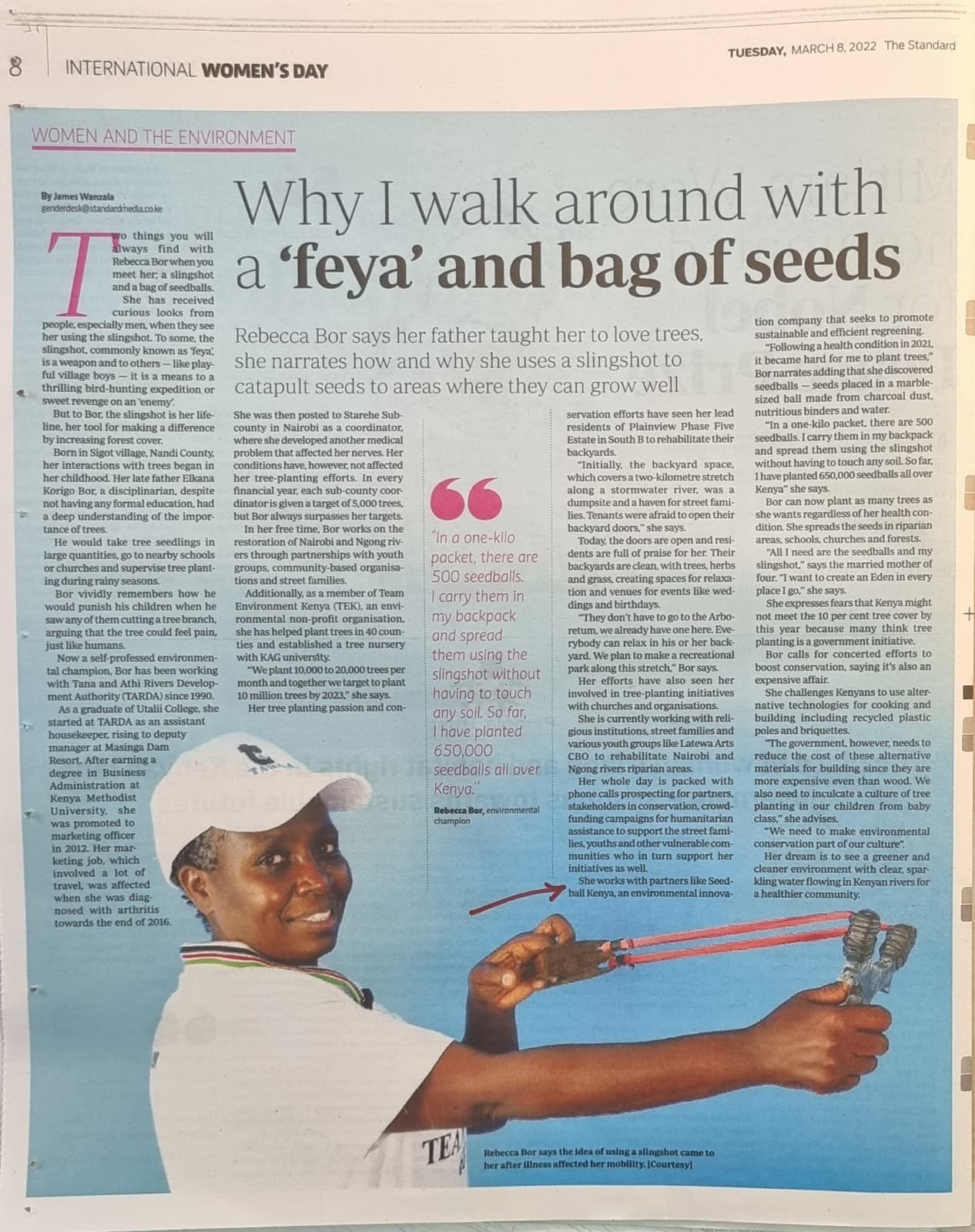The image is a full-page magazine article titled "Why I Walk Around with a Faya and Bag of Seeds" and focuses on International Women's Day. The article, written by James Wanzala, features a detailed caption describing the scene as well as the theme of Women and the Environment, which is highlighted in pink, underlined, and placed at the top left. The publication date, Tuesday, March 8, 2022, and the publisher, "The Standard," are shown at the top right in black font on a beige background. The page number, 8, is located at the top left.

The article background is a gradient of light blue, hosting four columns of text between which an inspirational quote in pink font is positioned: "In a one kilo packet, there are 5,000 seed balls. I carry them in my backpack and spread them using the slingshot without having to touch any soil. So far, I have planted 650,000 seed balls all over Kenya."

At the bottom of the article, a photograph showcases a smiling black woman, Rebecca Boer, who is depicted in a white short-sleeved polo shirt and a white baseball cap. She holds a slingshot in her right hand, pulling back the elastic band with her left. Her engaging, delighted expression underscores her commitment to environmental sustainability as she implements her father's teachings by using a slingshot to plant seeds across Kenya. Although the font is too small to read in detail, the headline and visible content strongly emphasize Rebecca's innovative approach to environmental conservation.